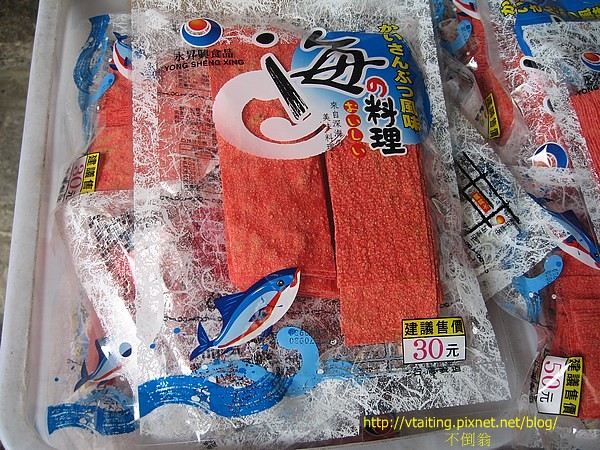The image depicts multiple packages of seafood, each packaged in clear plastic and stacked in a rectangular white plastic bin, dirtied to a gray in several spots due to wear. Each package features a vibrant design, with a prominent red sun at the top left, a blue crescent moon beneath it, and the words "yongsheng song" further below, alongside Japanese lettering. Inside each package, there are what appear to be rectangular-shaped red items, possibly not fish but something related to seafood cuisine such as nori or similar ingredients. On the bottom left of the package, a colorful blue, white, and red fish graphic is depicted amid blue sea waves, while the bottom right displays the number "30" next to an Asian currency symbol. Imposed over the bottom right of the image is a URL, "http://vtaiting.pixnet.net/blog/", in yellow font, accompanied by three Asian characters. The overall setting appears to be a grocery store or similar market environment.